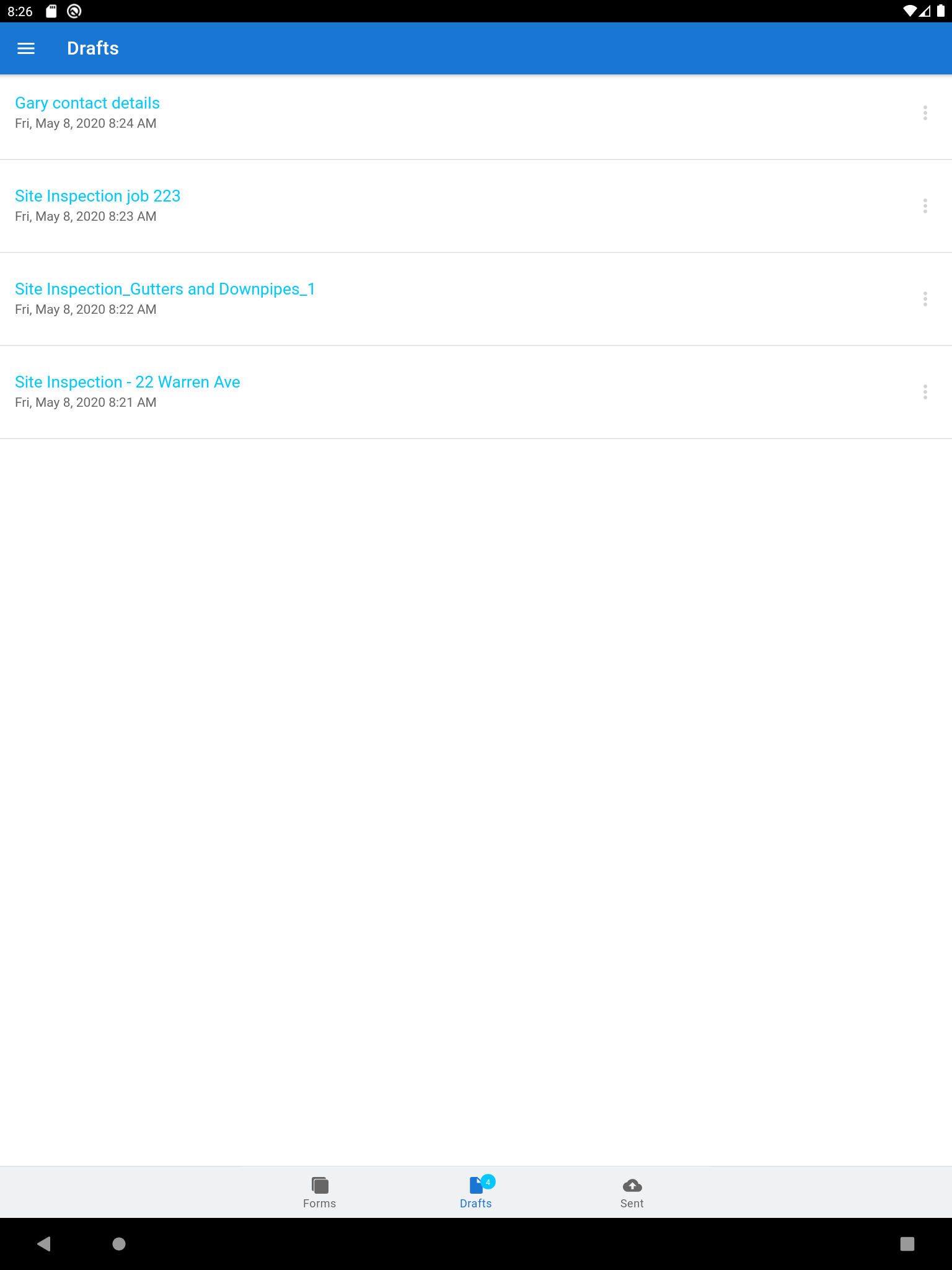This image displays a screenshot of the email drafts tab on a mobile device, possibly an iPad. At the very top, there is a black status bar featuring the battery percentage and WiFi signal indicators. Directly below, a blue header prominently displays the word "Drafts" on the left side, accompanied by an icon with three horizontal lines. 

The primary draft email listed is titled "Gary contact details" in light blue, with the corresponding date and time beneath it. Following this are three additional draft emails:

1. "Site inspection, job 223" with its date and time.
2. "Site inspection, gutters and downpipes one" dated Friday, May 8th, 2020, at 8:22 AM.
3. "Site inspection, 22 Warren Avenue" with its date and time.

At the bottom of the display, three small icons in the center, where the middle one is highlighted in blue, mark navigational shortcuts. Below these, a black bar provides quick access to device functions with icons for 'Go Back Home' and an option to minimize or maximize the screen.